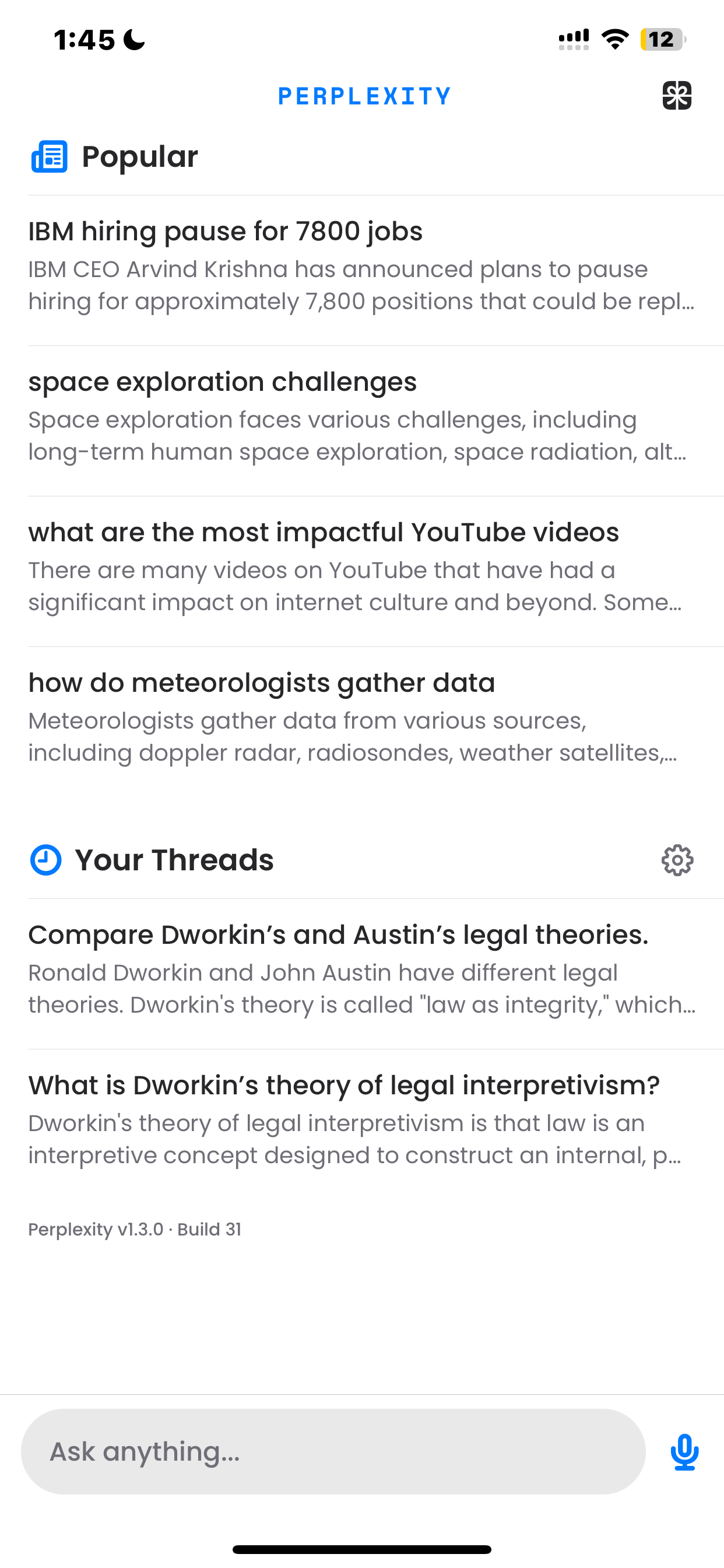The image depicts a cell phone screen displaying a website with various features and information. At the top, the phone's status bar shows a battery level of 12%, with a yellow icon on the left side. The phone has a good connection and is set to "Do Not Disturb," as indicated by a moon icon next to the time, which is 1:45.

In the main section of the screen, the text "Perplexity" is prominently displayed in blue. Below that, there's a "Popular" section featuring a blue image of some boxes. The headline reads, "IBM hiring pause for 7,800 jobs," detailing the company's announcement to halt hiring for approximately 7,800 positions. Additionally, there is a section on "Space exploration challenges," and another part discussing “What are the most impactful YouTube videos.”

Further down, information on “How do meteorologists gather data” is provided. Another section titled "Your Threads" includes a topic comparing "Dworkin's and Austin's legal theories," followed by a brief write-up discussing "What is Dworkin's theory of legal interpretivism."

At the bottom of the screen, there is an "Ask Anything" section with a gray space for input and a blue microphone icon next to it. The screen ends with a black bar underneath, presumably for navigation or submission purposes.